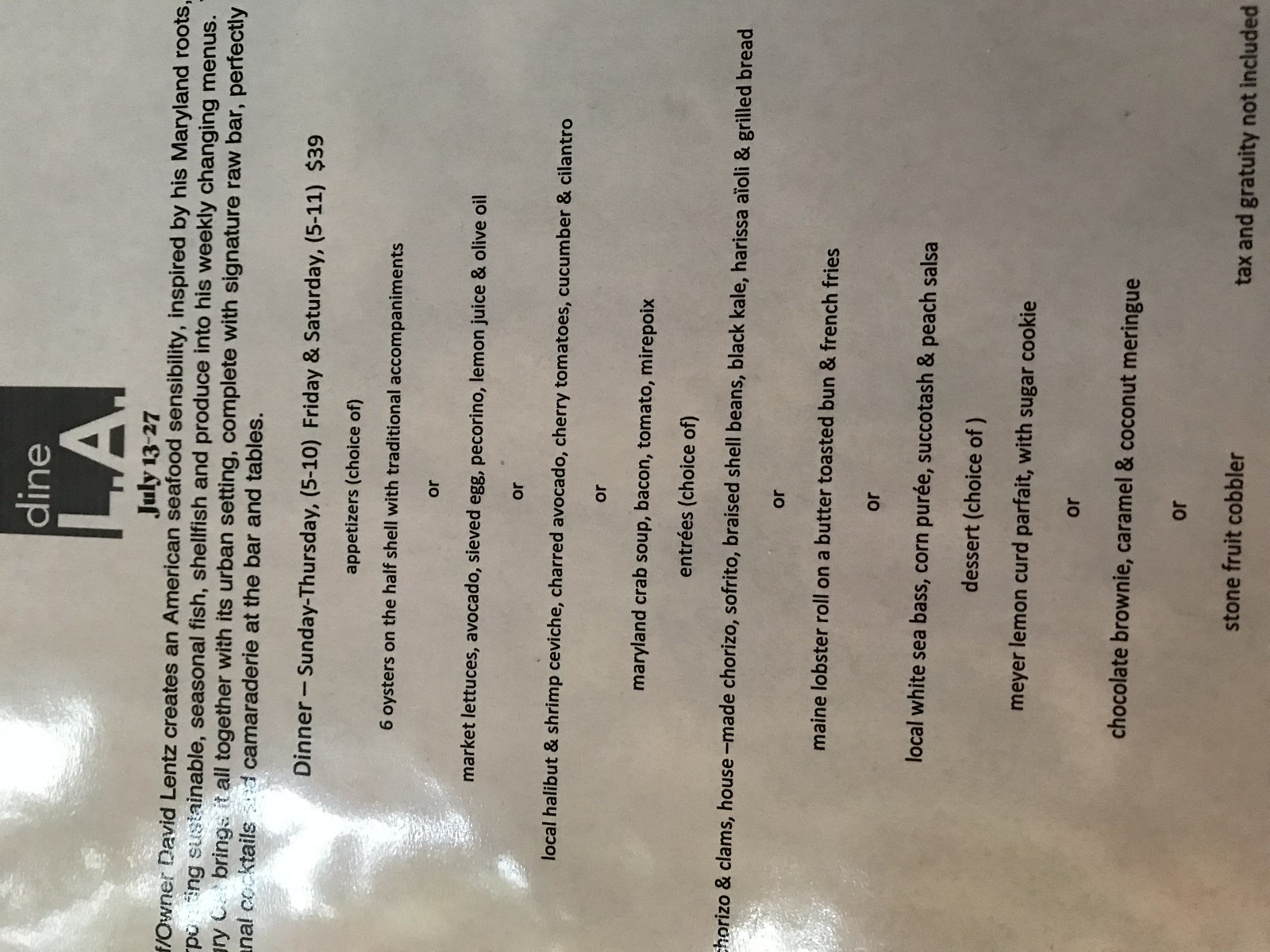The image depicts a laminated menu from "Dime LA" turned on its side, showcasing the offerings for the week of July 13th through the 27th. The menu highlights the culinary creations of Owner David Lentz, who integrates his Maryland roots into American seafood dishes, emphasizing sustainable and seasonal ingredients. The weekly rotating menu features an array of appetizers available for dinner from Sunday to Thursday. Some notable dishes include freshly shucked oysters, a market lettuce salad topped with avocado, egg, pecorino, lemon juice, and olive oil, a refreshing local halibut and shrimp ceviche, and a comforting Maryland crab soup. For dessert, there's a delectable stone fruit cobbler.